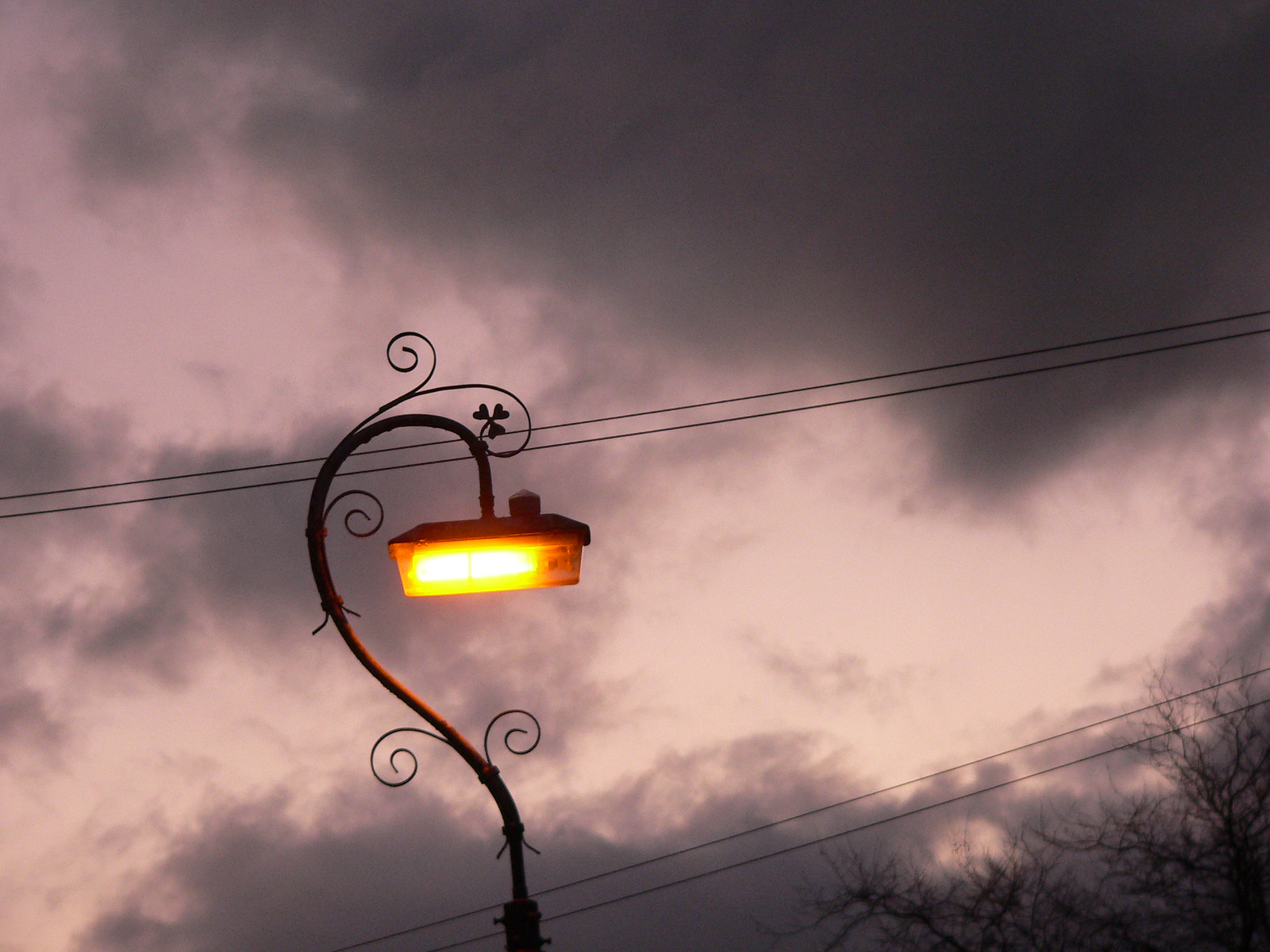The image features an ornate, curved lamppost with a floral theme, adorned with intricate tendrils and swirls that give it a decorative appearance. A prominent light fixture with a wide, flat, square shape hangs from the end of the curve, casting a yellowish-orange glow. The backdrop consists of power lines stretching horizontally from left to right. The sky behind these lines exhibits a dramatic gradient, transitioning from light purple to deep purple, with dark gray clouds adding to the contrast. In the bottom right corner, tree branches from distant trees protrude slightly into the frame.